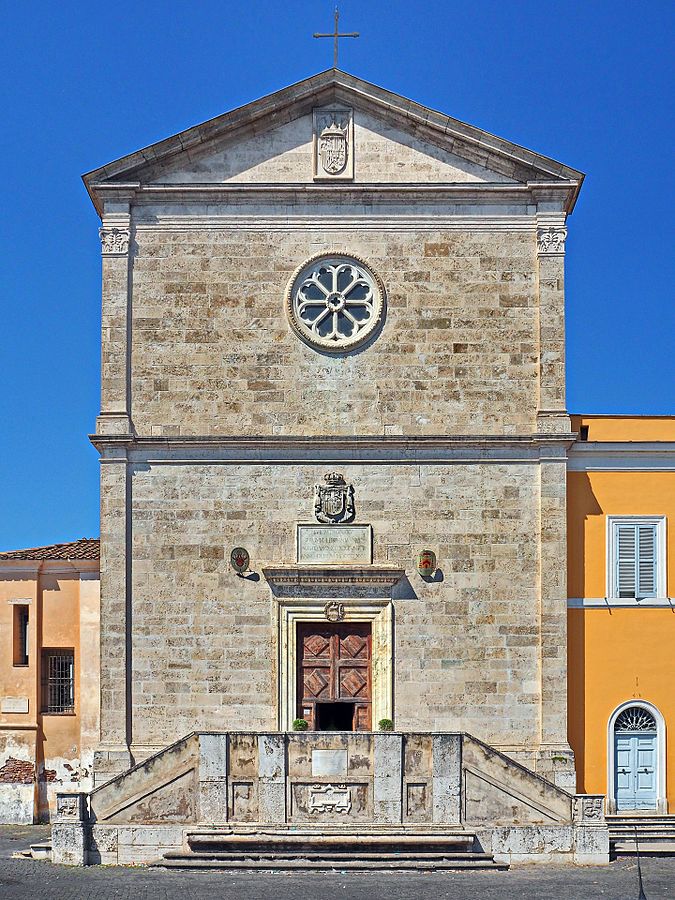This image captures the intricate front facade of the Church of San Pietro in Montorio, a majestic, light-colored stone edifice likely constructed from limestone. The structure features a peaked triangular roof crowned by a cross, beneath which sits a rectangular stone plaque. Centered prominently on the facade is a round stained glass window with eight distinct panels. Below the window, a coat of arms is displayed above a single, ornately decorated, dark brown wooden door. Flanking the door are two sconces, possibly serving as entry lamps. The stairway leading to the entrance splits to the right and left of the platform. Adjacent to the church, the attached structures are painted in deep golden hues. The right side displays an arched doorway with a shuttered window on the second story, while the left side consists of a smaller building with a tiled roof and wrought iron railings across the windows. The setting is completed by a dark-colored road in the foreground and a clear blue sky overhead, highlighting the architectural beauty of the scene.